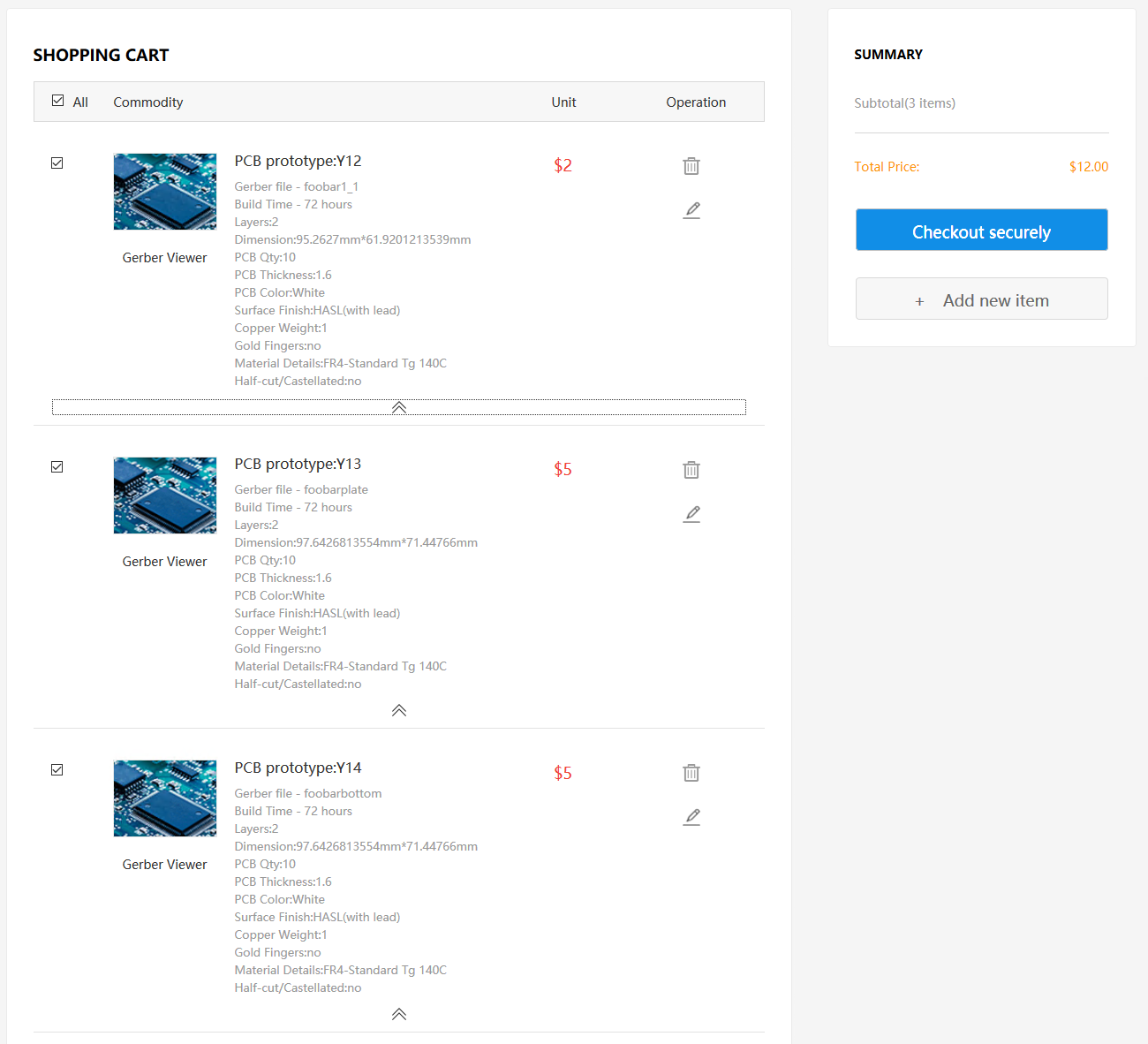The image depicts a computer screen with a light gray background showing a detailed view of a shopping cart for computer chips. The layout features a vertical panel on the right third of the screen. At the top of this panel, a white box labeled "Summary" in black letters is visible. Below this, "Subtotal (3 items)" is written in gray, followed by "Total Price: $12.00" in orange letters. Further down, a blue rectangular button with "Checkout Securely" in white letters is displayed, preceded by a light gray button labeled "Add New Item" in gray text.

Occupying the left two-thirds of the screen is a large white rectangle marked "Shopping Cart" in dark capital letters at the top left corner. A gray band runs along the top of this section, featuring various headings: a small white square with a checkmark labeled "All," followed by "Commodity," "Title," "Unit," and "Operation" headings.

Three individual panels display the selected items within the shopping cart. Each panel begins with a small check-marked square at the top left, indicating the selected status of the item. Each item has a rectangular color photograph of a computer chip, predominantly in blue and green hues. Below each image are the words "Gerber Viewer." To the right of each picture lies a detailed description of the item.

- The first item is labeled "PCB Prototype: Y12," followed by approximately ten additional lines of detailed information. The price is marked in red as "$2.00," with a trash can icon and a pencil icon for editing or removing the item to the far right.
- The second item follows the same structure and is labeled "PCB Prototype: Y13," priced at $5.00.
- The third item, similarly organized, is labeled "PCB Prototype: Y14," also priced at $5.00.

Overall, this image provides an orderly and comprehensive view of the items selected for purchase and pertinent options for managing the cart.